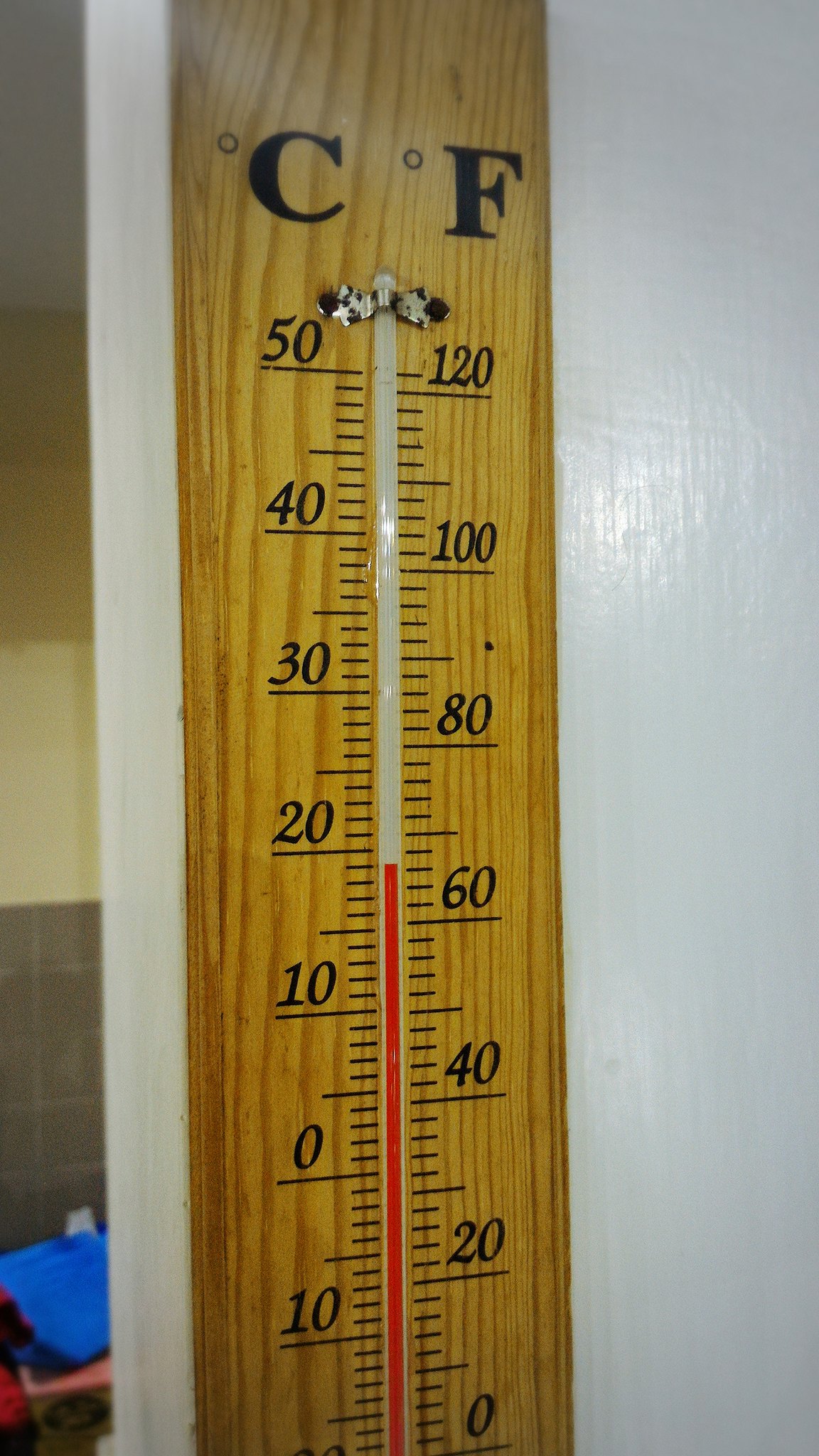In this image, a wooden thermometer is prominently featured, centrally located, and hanging on a white wooden wall. The thermometer is vertically oriented, extending from the bottom to the top of the frame. The main body of the thermometer is light brown, with a glass tube running through its center, partially filled with red liquid. Fahrenheit temperature readings are marked on the right side of the thermometer, starting from the bottom with 0, progressing upwards in increments of 20, and reaching 120 at the top. The letter "F" is visible at the top right. On the left side, Celsius measurements are displayed, beginning with -10 at the bottom, increasing by intervals of 10, and ending at 50 at the top, with the letter "C" at the top left.

The wall that the thermometer is mounted on dominates about 90% of the background, stretching from the right to the left of the image. On the left edge, approximately 10% of the frame reveals an adjacent room. The upper section of the wall in this room features a tan color, while the lower portion is darker gray with square tiles. Positioned on the floor in the bottom left corner is a box with a pink lid, on top of which a blue tile is resting flat. This setup provides a detailed context of the surrounding environment, emphasizing the contrast between the two rooms and highlighting the thermometer as the focal point.